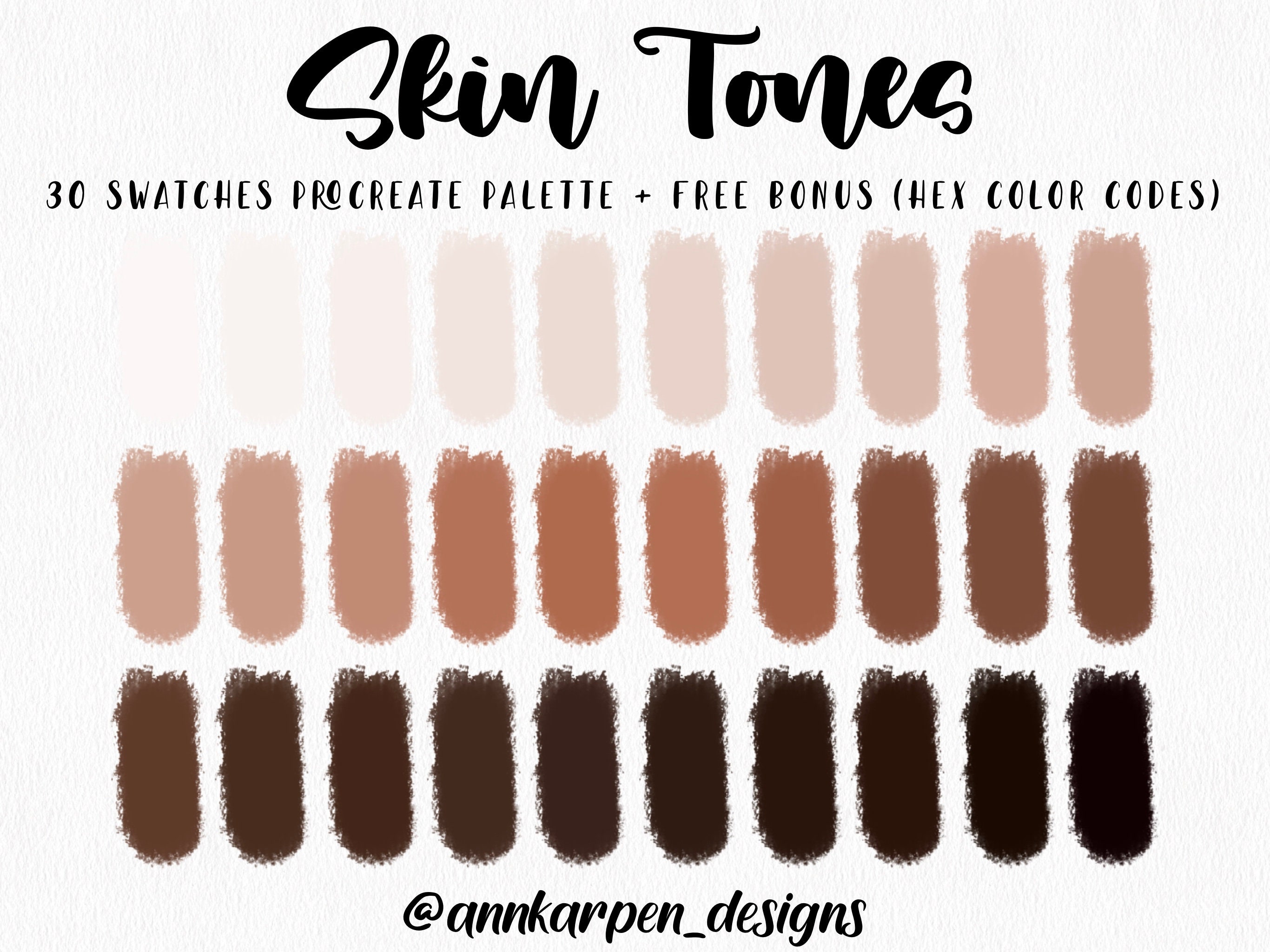The image depicts an infographic on skin tones, prominently featuring text at the top in large black font that reads "Skin Tones." Below this, a subtitle in a slightly smaller font states, "30 Swatches Procreate Palette + Free Bonus Hex Color Codes." The main section showcases an array of skin tone swatches arranged in three columns, starting from very pale white shades in the first row, moving to medium tones in the middle, and concluding with very dark black shades at the bottom. These color swatches stand out against an off-white, speckled background. At the bottom of the infographic, the social media handle "@AnneCarpin_designs" is displayed. This visual guide allows users to compare these tones for purposes such as matching makeup to their skin tone.